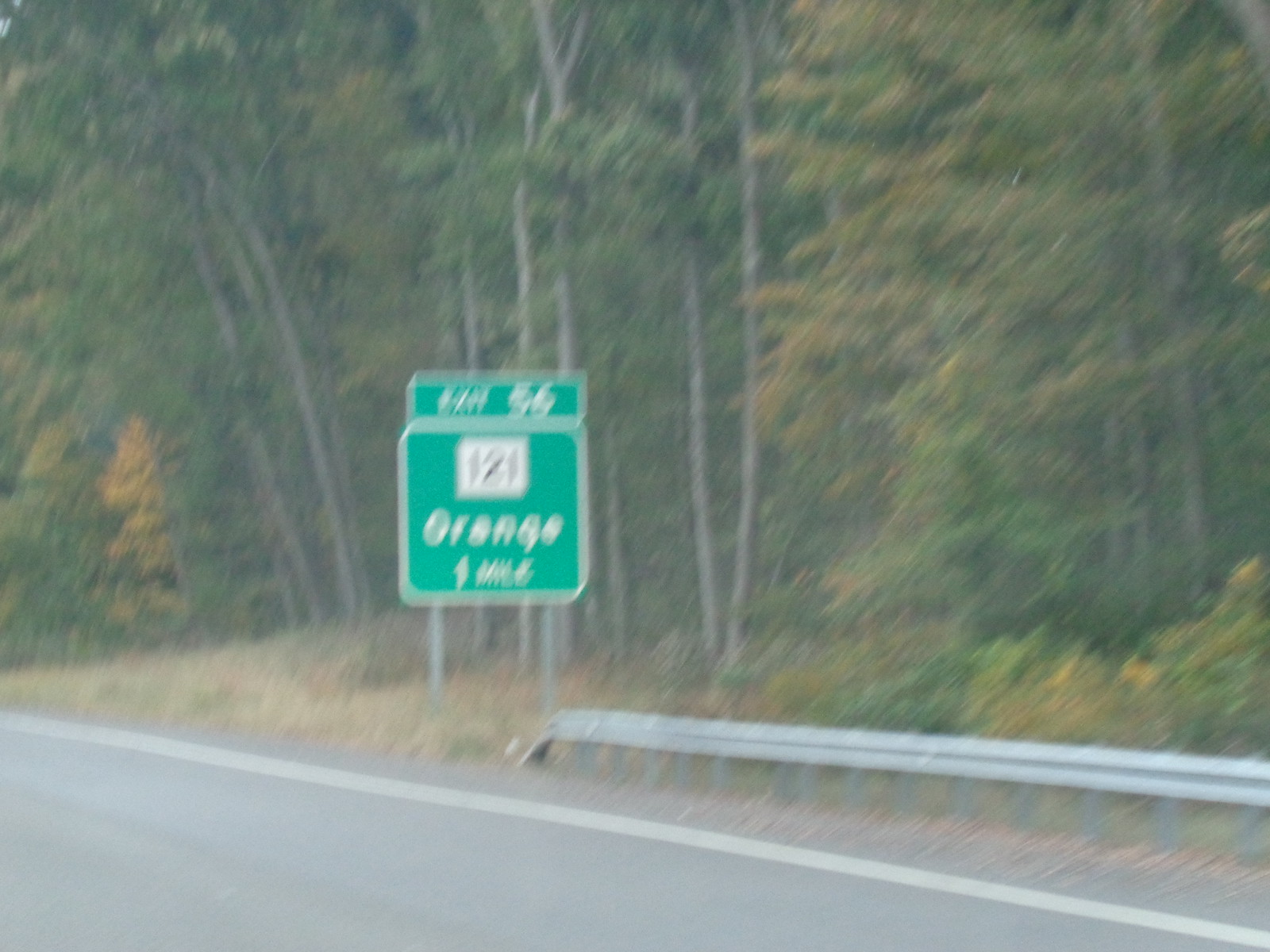A detailed road sign stands by the side of a gray road marked with a white stripe along its right edge. Adjacent to the road, a short metal railing supported by evenly spaced gray legs provides a barrier. The road sign itself is mounted on two gray poles and features a square shape bordered in white. At the top of the sign is a rectangle, also bordered in white, displaying the numbers "56" or "55." Below this, the sign reads "121 Elgin O'Grange, 1 male" in white lettering, with the number "121" prominently in black. Behind the sign, a line of tall, slender trees with green foliage is interspersed with some trees showcasing vibrant autumn hues of brown and red.